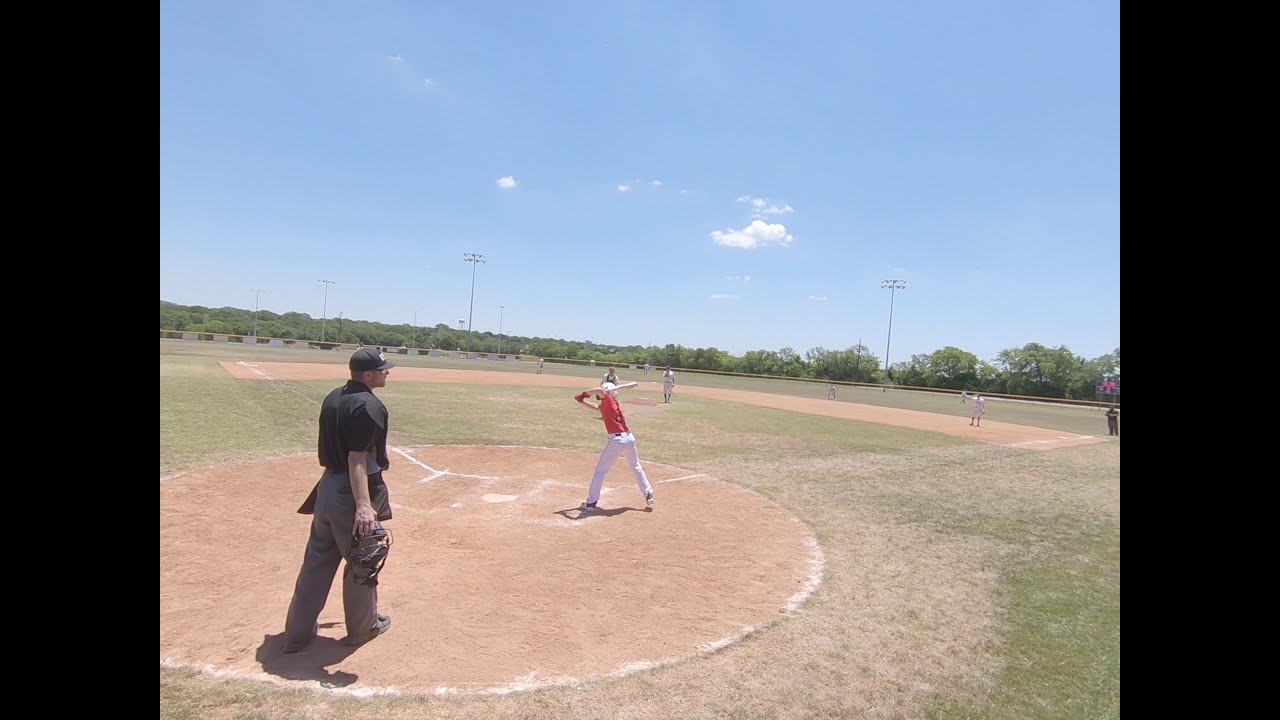The photograph captures a vibrant scene of a baseball diamond on a clear day. In the center, a young batter, perhaps around 10 years old, stands poised to swing, wearing white baseball pants and a red shirt. Behind him, the umpire, dressed in a black shirt, hat, and gray khakis, holds a catcher's mitt or mask. They stand on a dirt-filled chalk ring, with the lush green grass of the field extending beyond. Scattered across the outfield are other players in white uniforms, indicating defensive positions. Surrounding the field is a boundary fence, with rows of tall, green trees beyond it. Towering over the scene are two large stadium lights, one on the left and one on the right, with a hazy blue sky dotted with a few white, puffy clouds overhead. The setting exudes a sense of a well-maintained and lively baseball game, likely a youth match, with an atmosphere that balances competition and camaraderie.